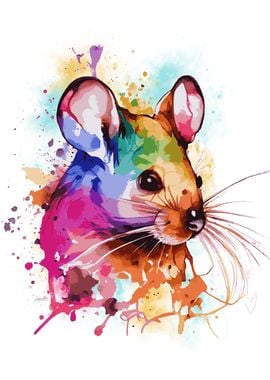This image is a vibrant watercolor painting of a mouse, depicted with a rich array of colors and intricate details. The mouse is positioned in profile, facing towards the right side, with the right side of its face and shoulder area prominently displayed. Its body is an amalgamation of pink, purple, yellow, and green hues. The ears are a striking blend of pink, orange, red, white, and purple, which contrast the black nose and lush whiskers in shades of orange and purple. The mouse's lively black eyes add character to its expressive face.

The background consists of a soothing palette of blues and yellows, creating a harmonious setting for the mouse. Adding a touch of whimsy, a small red heart is seen in the corner of the painting. The artwork is characterized by splashes of color throughout, with splatter effects in magentas, teal, and green scattered both on and around the mouse, giving the impression that the mouse is dissolving into the portrait. The overall composition is dynamic and engaging, drawing the eye to both the intricate details and the vibrant bursts of color.